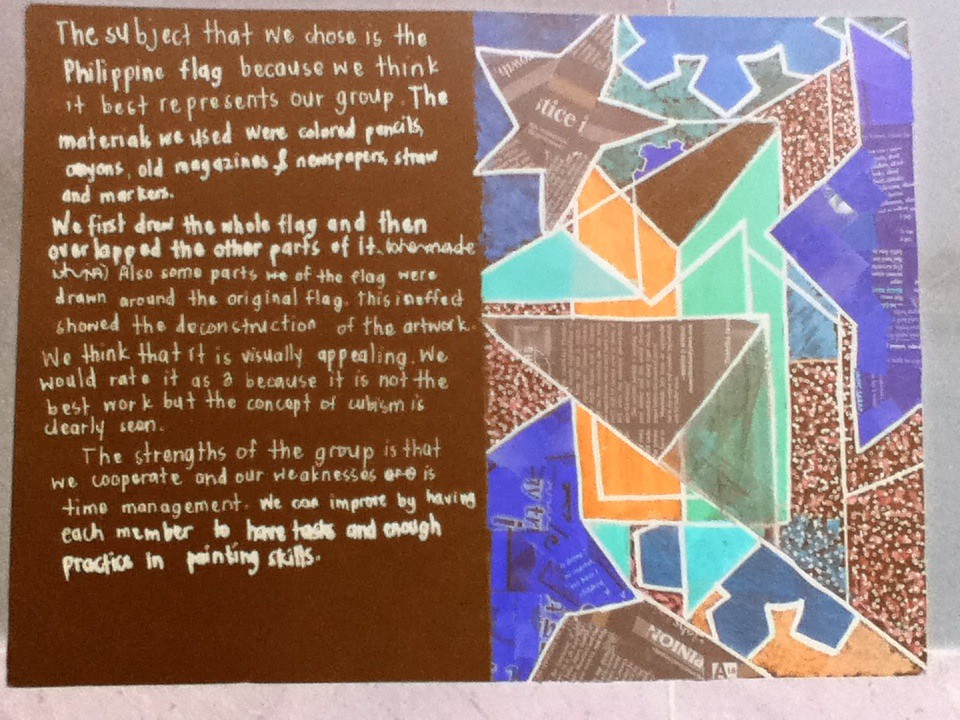The image showcases a handcrafted poster that prominently features a collage and accompanying text. On the left side, the text is written on a brown background in a mix of bold and regular white handwritten letters. Some parts are thicker while others are thinner, creating a slightly uneven but distinct look. This text explains that the group selected the Philippine flag to best represent them and describes the mixed materials they used, including colored pencils, crayons, old magazines, newspapers, straw, and markers. On the right side of the poster, a visually captivating collage incorporates various geometric shapes and snippets of newspapers in an abstract style. The collage predominantly features a color palette of brown, blue, green, and orange with white borders. Despite its intricate detail and small, difficult-to-read text, the collage remains central to the composition, with almost no background visible, emphasizing a hands-on, artistic style reminiscent of children's artwork.